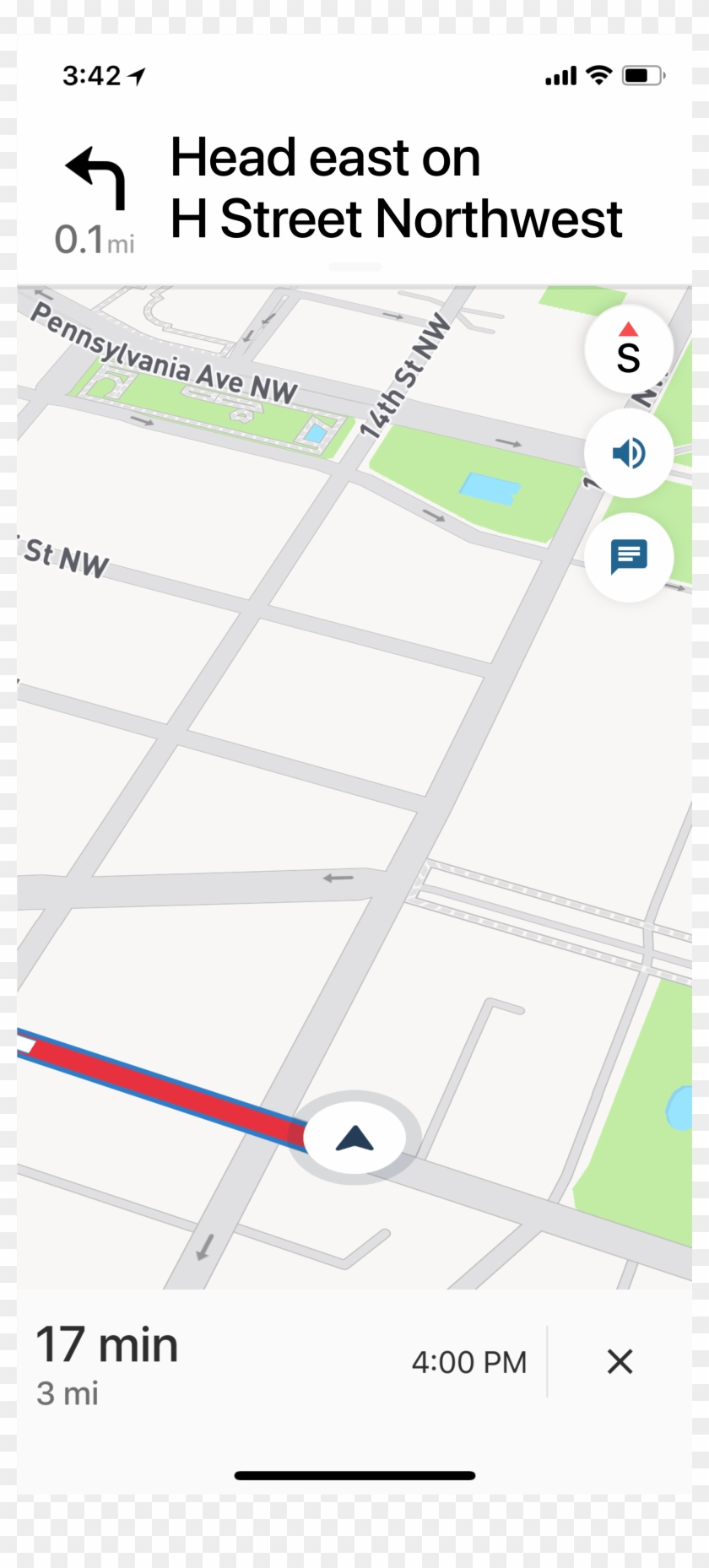This image, captured on a smartphone, displays a digital map of the District of Columbia. The map is encased in a checkered border. At the top, there is a time stamp showing 3:42 PM alongside a send arrow, a Wi-Fi icon, and a battery icon, all within a white section. Directly below, a left-facing arrow indicates that the user is to travel 0.1 miles east on H Street Northwest. 

The map prominently features landmarks such as Pennsylvania Avenue Northwest and 14th Street Northwest. Various icons related to street navigation, sound, and text messaging are visible on the map interface. Below these icons, the map provides additional information: an estimated travel time of 17 minutes, a distance of 3 miles, and the current time of 4 PM. To the right, there is a closeout 'X' button, and at the bottom, a home button is present.

The user’s current location is not distinctly marked, making it unclear exactly where they are starting from. Although Pennsylvania Avenue Northwest and 14th Street Northwest are easily identifiable, another cross street's name is obscured by the icons at the top of the screen.